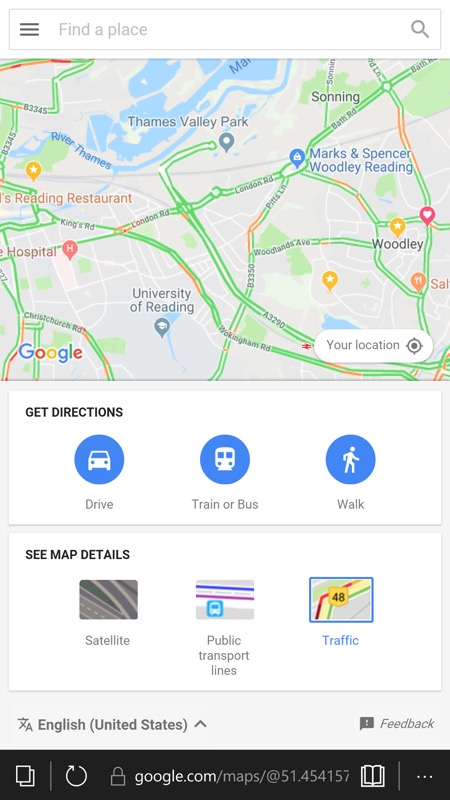A person is using a smartphone to access Google Maps. They are specifically viewing the general traffic conditions in an area, without selecting any particular route or mode of transportation. On the bottom of the screen, the 'Get Direction' options for driving, taking the train or bus, and walking are visible but not chosen. Instead, the user has activated the 'See Map Details' option and highlighted the traffic layer. As a result, the streets on the map are color-coded according to traffic conditions: green indicates smooth flow, yellow points to moderate traffic, and red signifies heavy congestion. Notable landmarks around the area include a hospital, a university, a park, and a place called Marks and Spencer Woodley Reading. The map also features Thames Valley Park and the River Thames, suggesting the location is in or near London, England.